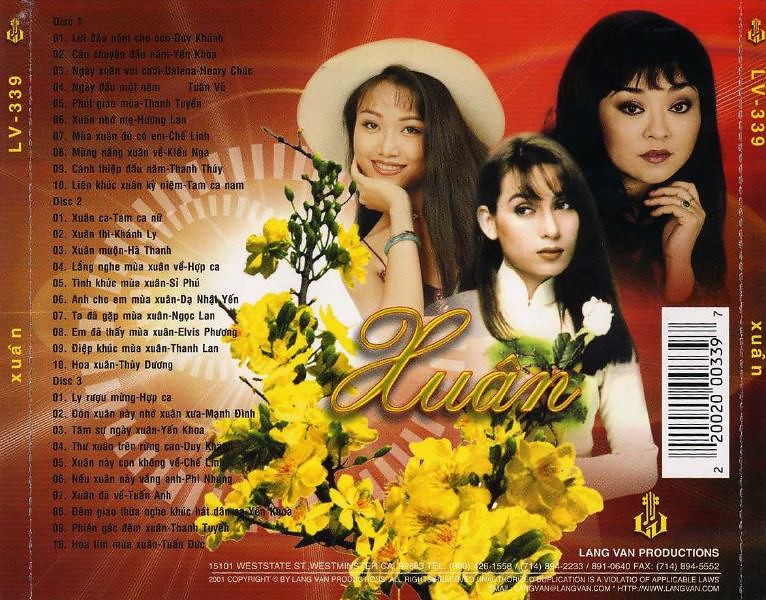The back cover of this CD, predominantly red with a yellow floral design in the center, features text written in an Asian language. It showcases an image of three Asian women. One woman, wearing a hat and a jade bracelet, rests her head on her chin. Another woman, her lips painted red and wearing a small ring, also supports her chin with her hand. The third woman, adorned in a traditional white dress with a high collar, holds a single white rose. In addition to the barcode on the right-hand side, the cover lists the songs spread across three discs, each containing 10 tracks.